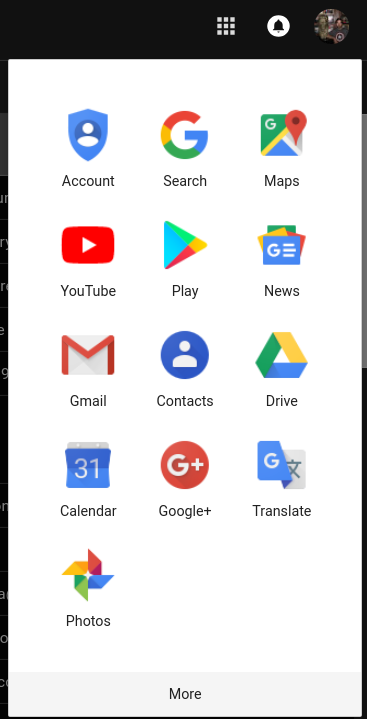The image is a screenshot from a website, likely taken on a smartphone. At the top of the screen, there is a black banner spanning the width of the device. The left border of the screen is thicker than the right border. Near the top, there is a small white square composed of three smaller white squares arranged vertically. Below this, there is a round icon featuring a black ball, followed by another circular icon displaying a user's image.

The main background of the screen is white, featuring several icons arranged in a grid of three columns. The top row of icons includes "Account," "Search," and "Maps." The second row features "YouTube," "Play," and "News." The third row shows "Gmail," "Contacts," and "Drive," followed by the fourth row with "Calendar," "Google Translate," and "Photos." 

At the bottom of the screen, there is a very thin black line. Below the white background with the icons, there is a light gray banner. In the center of this banner, the word "More" is displayed, with the "M" capitalized and the rest of the letters in lowercase, though the description appears to have a typo in the last letters ("o-r-d-p").